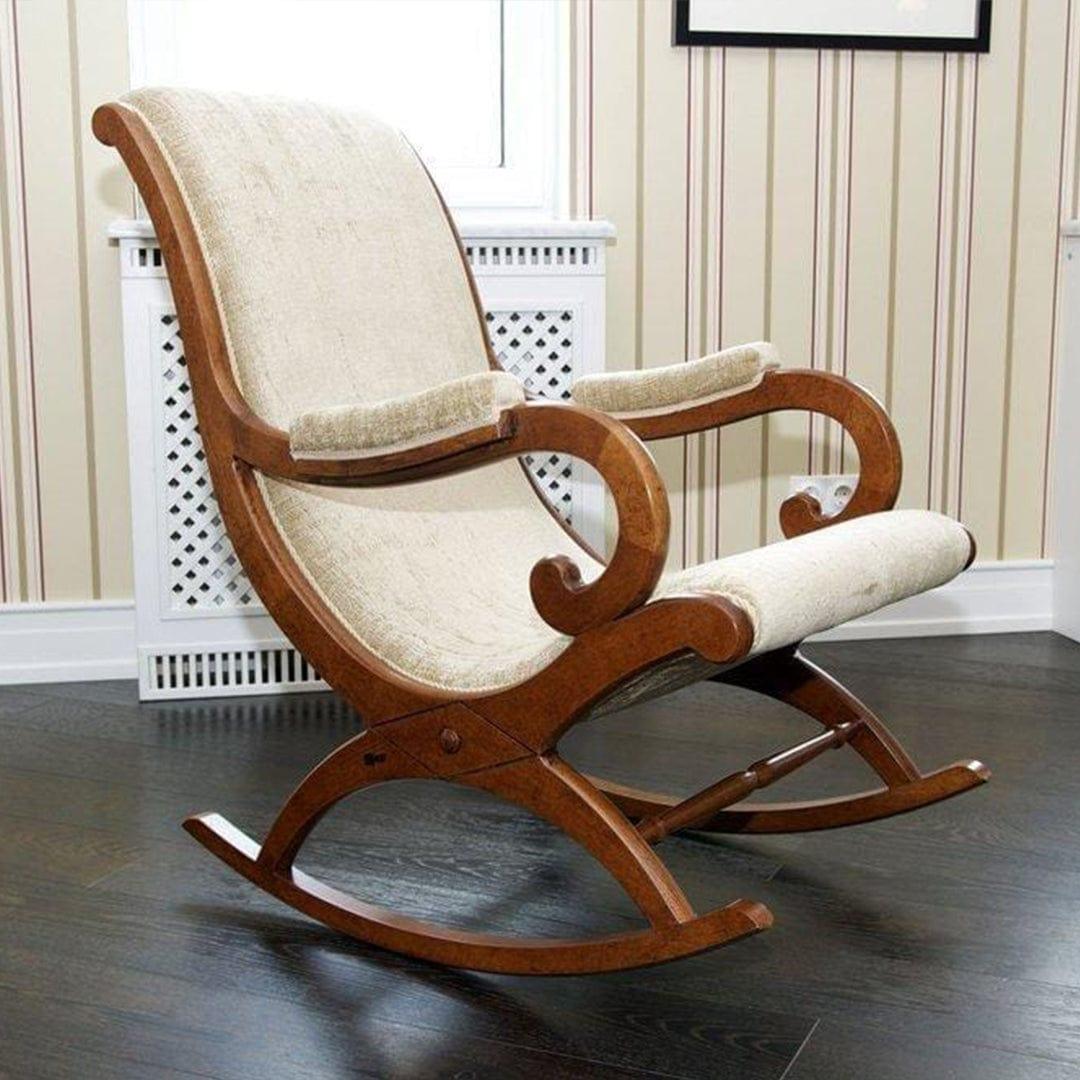In this photograph, a wooden rocking chair with a dark brown frame is prominently featured. The chair is covered with soft, white cushions that extend from the top of the high backrest down to the rounded seat, as well as on the armrests. It is positioned at an angle, slightly turned to the right, on a dark wood floor. Behind the rocking chair, the walls are adorned with wallpaper featuring a muted lattice pattern in pale colors, incorporating shades of light yellowish, green, and faint red. A white, old-style heating device with small vent holes sits directly behind the chair, topped off with a window. The overall scene captures a cozy and inviting corner of a home.